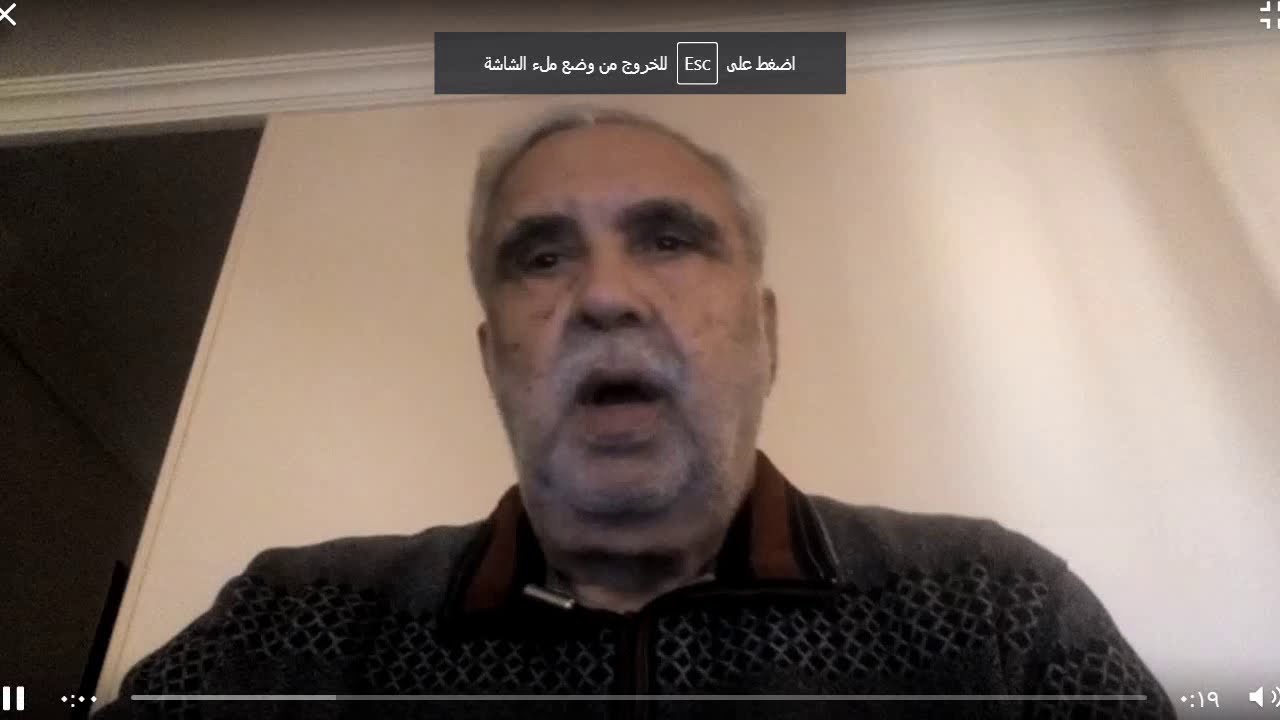This horizontal rectangular image appears to be a paused frame from a video clip or possibly a Zoom call, as indicated by video control icons located at the bottom of the screen, including a pause button, a progress bar, and a volume icon. In the center of the image is an elderly man, likely in his 60s or 70s, with gray hair, a light gray mustache, and a light goatee. He is facing forward and has his mouth open, suggesting he was in the middle of speaking when the image was captured. The man is wearing a polo shirt that features a diamond-shaped pattern with gray outlines on a dark background. The collar of the shirt is accented with alternating black and dark brown stripes. The background consists of a beige-colored wall with white crown molding at the top, and a doorway is visible to the far left, leading into another room. The image is framed with some interface elements, such as an X in the top left, a full-screen icon in the top right, and foreign language phrasing mid-screen, suggesting an application or platform with multiple language support.